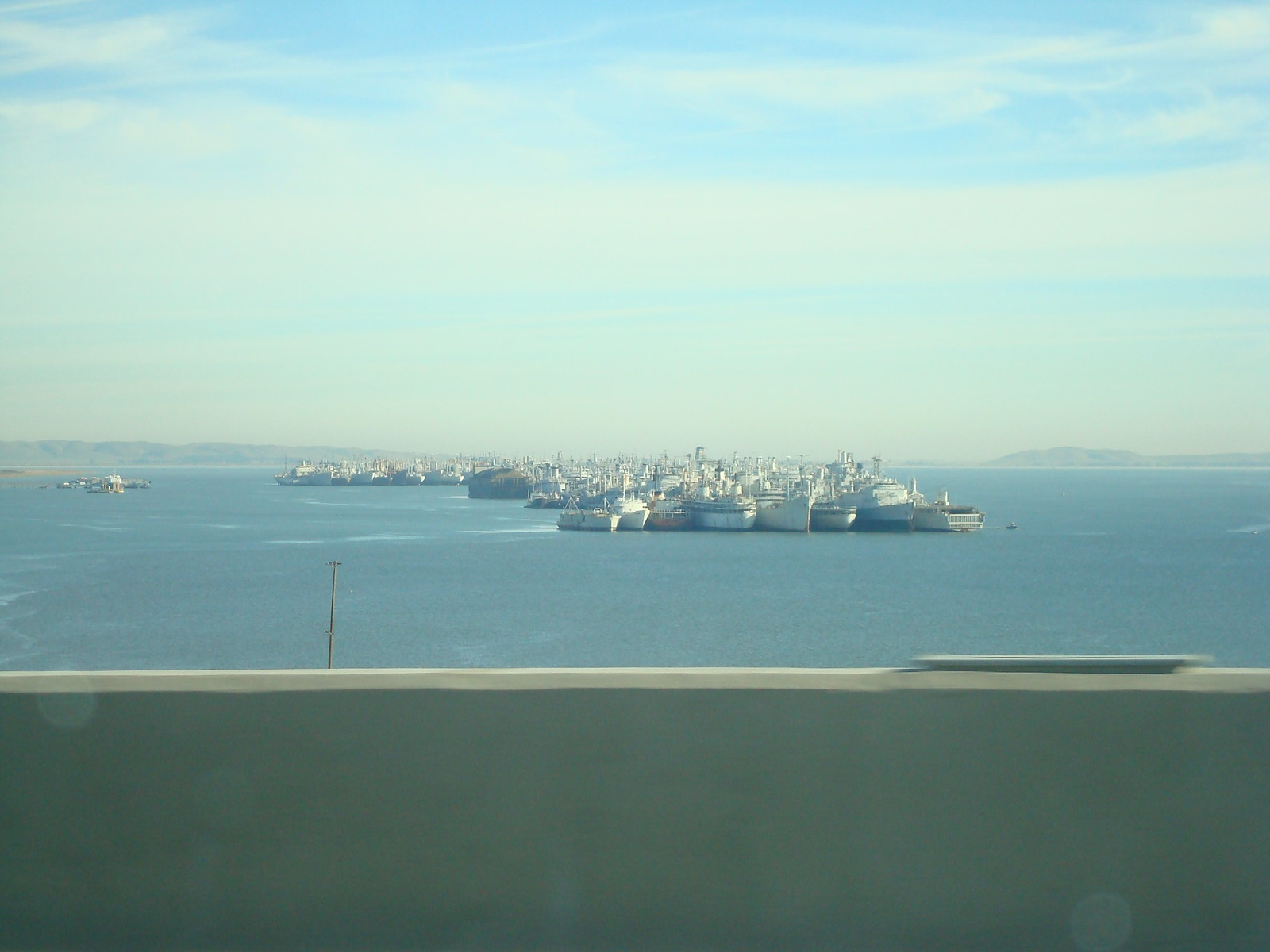This image captures a scenic aerial view taken from a balcony or a position high above a large, serene body of water. The foreground reveals a ledge with verdant greenery, possibly part of a nearby balcony or boat. The central focus of the scene is a substantial collection of boats clustered together in the calm, expansive water, which reflects various shades of blue indicating different depths. These boats, both large and small, are densely packed, indicating they might be docked or in a salvage yard.

Flanking the edges of the image, two shallow mountain ranges emerge on the horizon; one on the right is silhouetted against a clear blue sky with light clouds, and the other on the left offers a mirrored outline. The overall setting is outdoors, likely captured in the middle of the day, with natural colors like green, blue, white, gray, tan, black, and silver prominently featured. The tranquil waters stretch out to meet the horizon where the boats and distant land converge, creating a picturesque scene abundant with natural beauty.